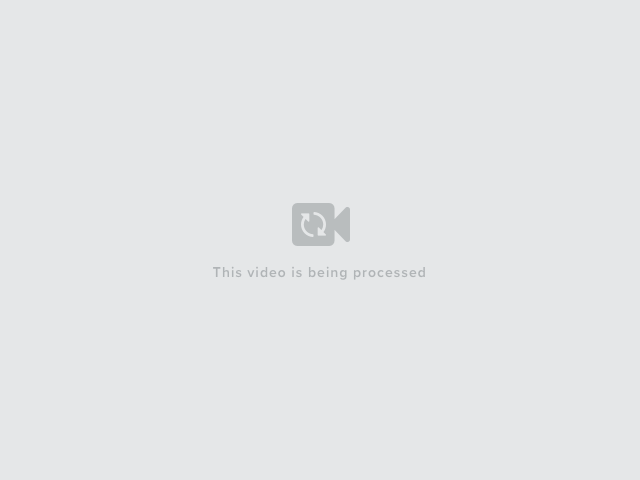The image is an almost square, light gray rectangle, very slightly wider than it is tall. At the center is a dark gray illustration resembling a TV camera, composed of a square atop a left-tilted triangle, with another small square on the left side of the triangle. Inside the camera image, there is a white refresh arrow symbol, which consists of a line that starts from the bottom, curves upward to form a small triangle, and then continues to make a nearly complete circular shape with another small triangular arrowhead. Below this camera illustration is light gray text that reads "This video is being processed," centered directly beneath the image. The background is plain light gray, ensuring a clear contrast with the darker camera illustration and the accompanying text.